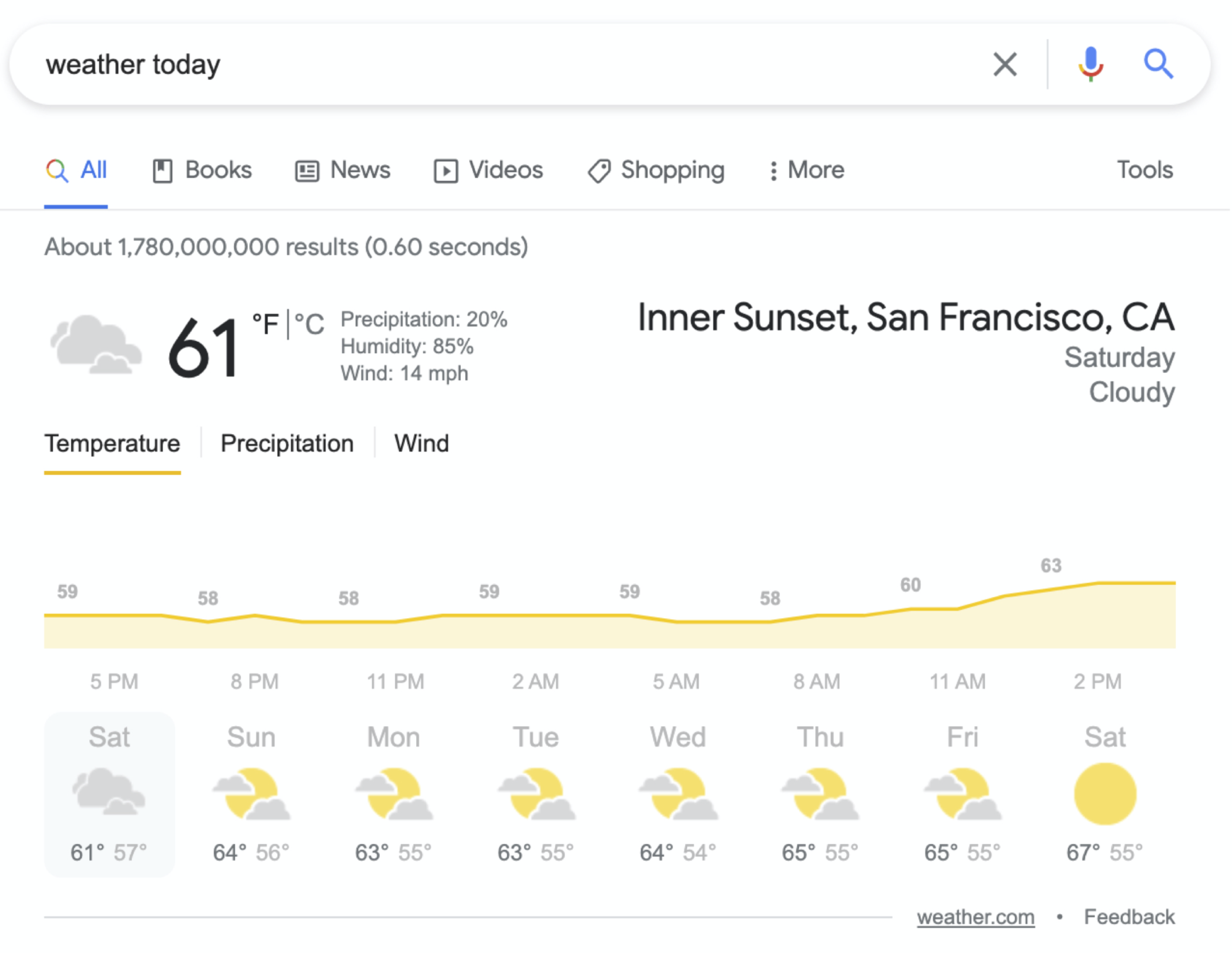The image depicts a Google search results page for "weather today." At the top, there is a prominent oval search bar with a white background and a subtle gray shadow. In the left section of the search bar, the query "weather today" is displayed in a small, black Sans Serif font. On the far right, a gray 'X' icon is present, followed by a faint gray divider line. Next to the divider on the right, there is a microphone icon with a blue speaker. The lower part of the microphone is a gradient from orange on the left to red on the right, with a blue stand. Adjacent to this is a blue magnifying glass icon.

Below the search bar, the navigation menu is visible. The first option, "All," is highlighted with a bold blue underline indicating it is selected, and is accompanied by a multicolored magnifying glass in Google's colors. Other menu options are displayed in gray: "Books" with a book icon featuring a top-left bookmark, "News" with a newspaper icon, "Videos" with a play button icon, "Shopping" with a price tag icon with a central dot, and "More" with a stack of three circular icons. On the far right, there's a "Tools" option.

Under the menu, a light gray line divider separates the menu from the search results. Below this divider, small gray text in Arial font indicates there are "About 1,780,000,000 results (0.60 seconds)." Further down, in larger black text, the location "INNER SUNSET, SAN FRANCISCO, CA" is specified. In smaller gray text beneath, the day "Saturday" and the weather "Cloudy" are indicated.